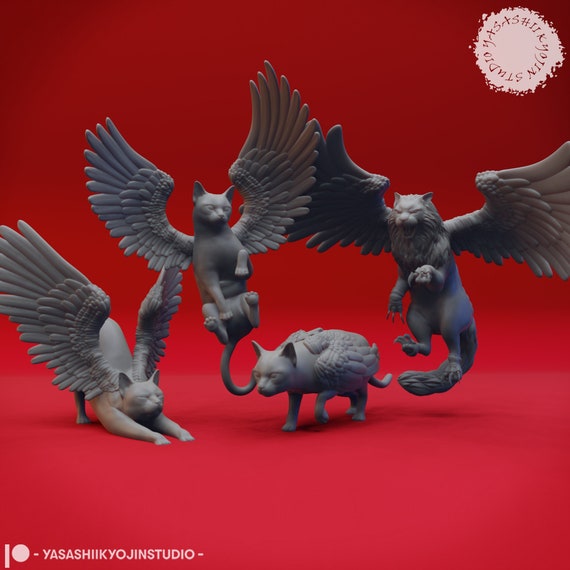In the image, four winged, cat-like creatures are prominently displayed against a vivid red background. Three of these creatures are hovering in mid-air with their expansive wings fully extended, showcasing their flight capabilities. One of the airborne creatures on the right appears particularly fierce, with a ferocious mane around its head and claws extended, suggesting it might be more like a lion. The creature in the center of the aerial trio seems to be moving away, while the one on the left is in the process of landing, stretching its wings high. Below them, the fourth creature stands on the ground, its belly visible towards the viewer and wings spread out. The overall color scheme is dominated by shades of gray for the creatures, contrasted sharply by the red background, with additional tones of black, white, and off-white. On the top right corner, the logo of an entity, possibly the studio's branding, is present. Meanwhile, in the bottom left corner, white text reads "YASASHIKYO JIN STUDIO," indicating the studio behind this intriguing image. This detailed digital creation captures a dynamic scene of these mythical, winged animals in motion, framed within a strikingly bold backdrop.